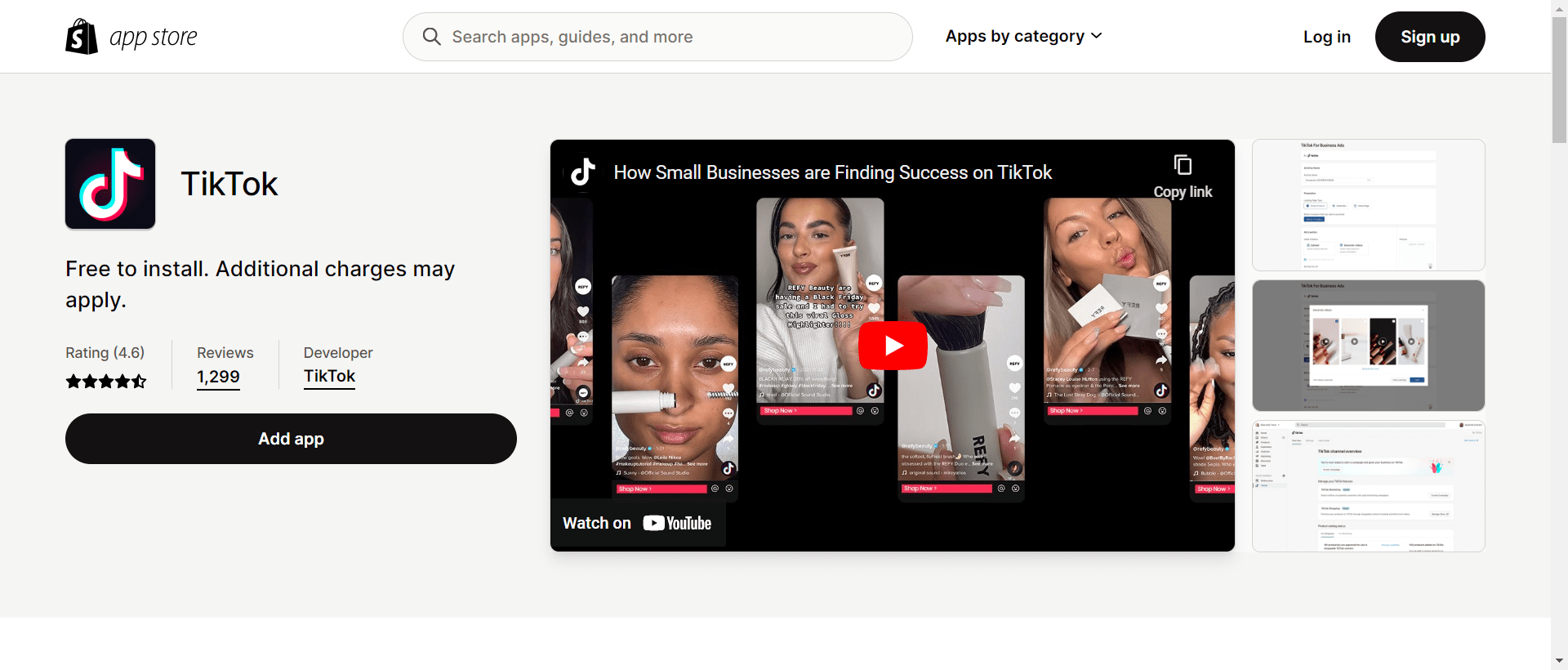A colorful landscape screenshot capturing a user's laptop screen while browsing an app store. The app store interface prominently displays its distinctive logo, an 'S' emblazoned on a black background, followed by the text "App Store" in bold uppercase letters. 

Dominating the screen is a feature listing for TikTok, showcasing its recognizable logo. The listing indicates that TikTok is free to install, though additional charges may apply. It boasts a high rating of 4.6 stars based on 1,299 reviews. The developer is noted as TikTok, and users are prompted to add the app via a conspicuous large black button with white text.

A promotional video highlight advertises the successes small businesses can achieve on TikTok, ready to be played. Above this central section, a navigation bar includes a search field labeled "Search apps, guides, and more." Next to it is a drop-down labeled "Apps by Category," hinting at further classifications available within the store. The navigation bar concludes with options for logging in and signing up, providing clear entry points for user interaction.